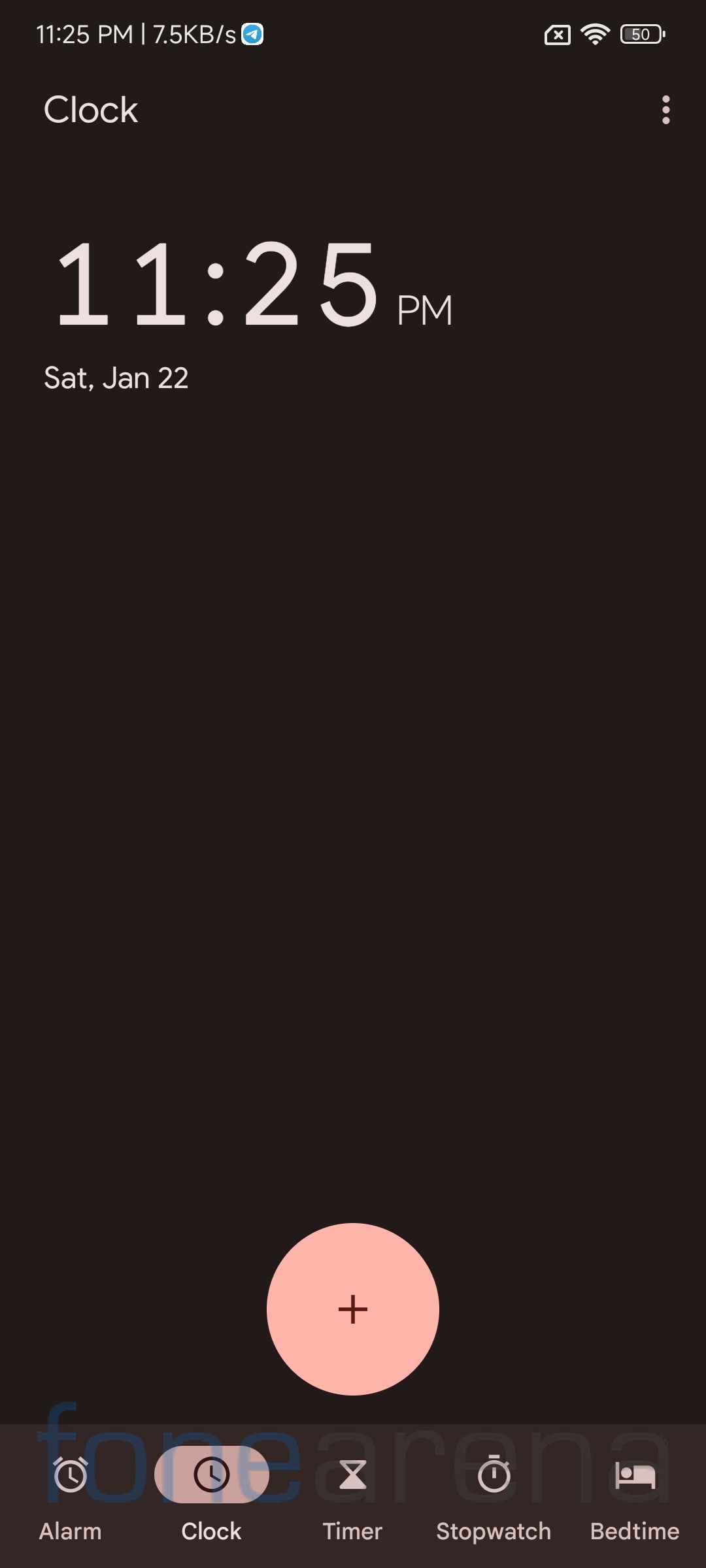The image depicts a mobile device screen with a black background. At the top of the screen, the time is displayed as 11:25 PM. Additionally, the screen shows a data speed of 7.5 KB/s, a Wi-Fi icon, and a battery indicator which is approximately three-quarters full.

Below the time display, there is the word "Clock" and a vertical ellipsis (three dots) positioned on the right side. Beneath this, the date and time are reiterated as "11:25 PM, Saturday, January 22nd." A large portion of the lower area in the image is empty space.

Towards the bottom, there is a pink oval with a plus (+) sign in the center. Underneath this oval, the text reads "Alarm, Clock, Timer, Stopwatch, and Bedtime." Each of these options is accompanied by its respective icon: an alarm clock for the "Alarm," a clock for the "Clock," an hourglass for the "Timer," a stopwatch for the "Stopwatch," and a bed for the "Bedtime."

In the top left corner, there is a light blue box, though its purpose isn't clear. The rest of the screen appears blurry, and there seems to be some text at the bottom that is illegible, possibly indicating something about the phone, but it is unreadable.